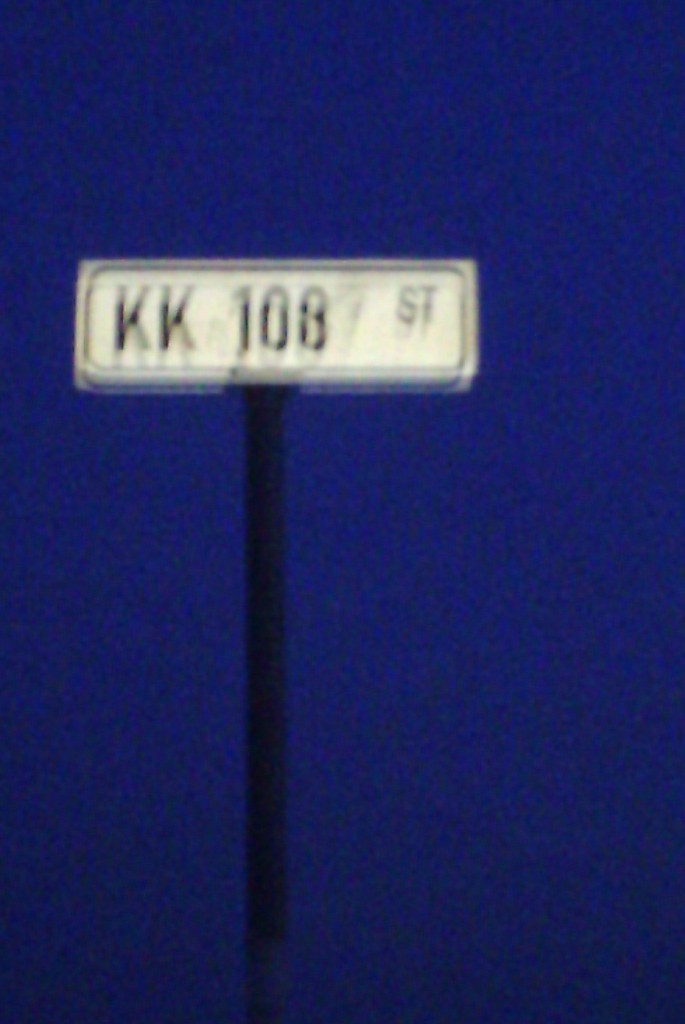This is a blurry nighttime photograph featuring a black metal pole positioned towards the middle left of the image. The pole supports a rectangular white street sign framed with a black border, and bears the text "KK 108th Street" in black lettering. The background is a dark, indigo-blue night sky. The pole appears dark blue at the bottom and black towards the top, due to the nighttime lighting. The image's dimensions are taller than it is wide, and it contains no people, animals, plants, buildings, vehicles, birds, or water. The simplicity and lack of additional elements suggest a clear focus on the street sign and its immediate surroundings.